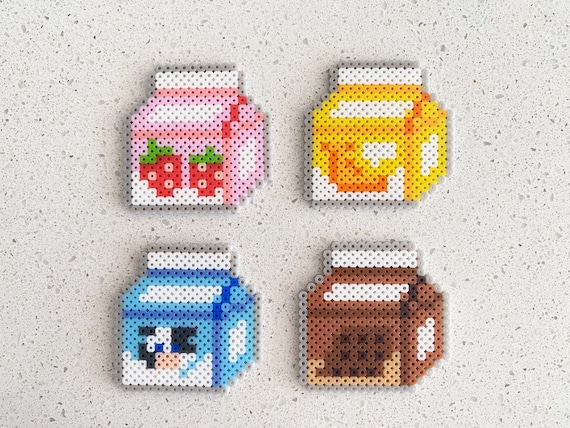The image portrays a top-down view of a white marble kitchen countertop adorned with grey, light, and dark specks. Centered in a grid-like pattern, 2x2, are four distinct, small milk carton art projects made from colorful plastic beads, typically used in children's modeling activities where beads are arranged and fused together. The top left carton is pink, featuring two red strawberries with green tops. Adjacent to it in the top right, a yellow carton showcases an orange semi-circle with surrounding white and orange specks. The bottom left carton is blue, depicting a cow's head in black with white and pink details. Finally, the bottom right carton is brown, resembling a chocolate bar with dark brown squares arranged in a grid pattern. Each carton is intricately designed, presenting a playful and vibrant scene against the sophisticated stone background.